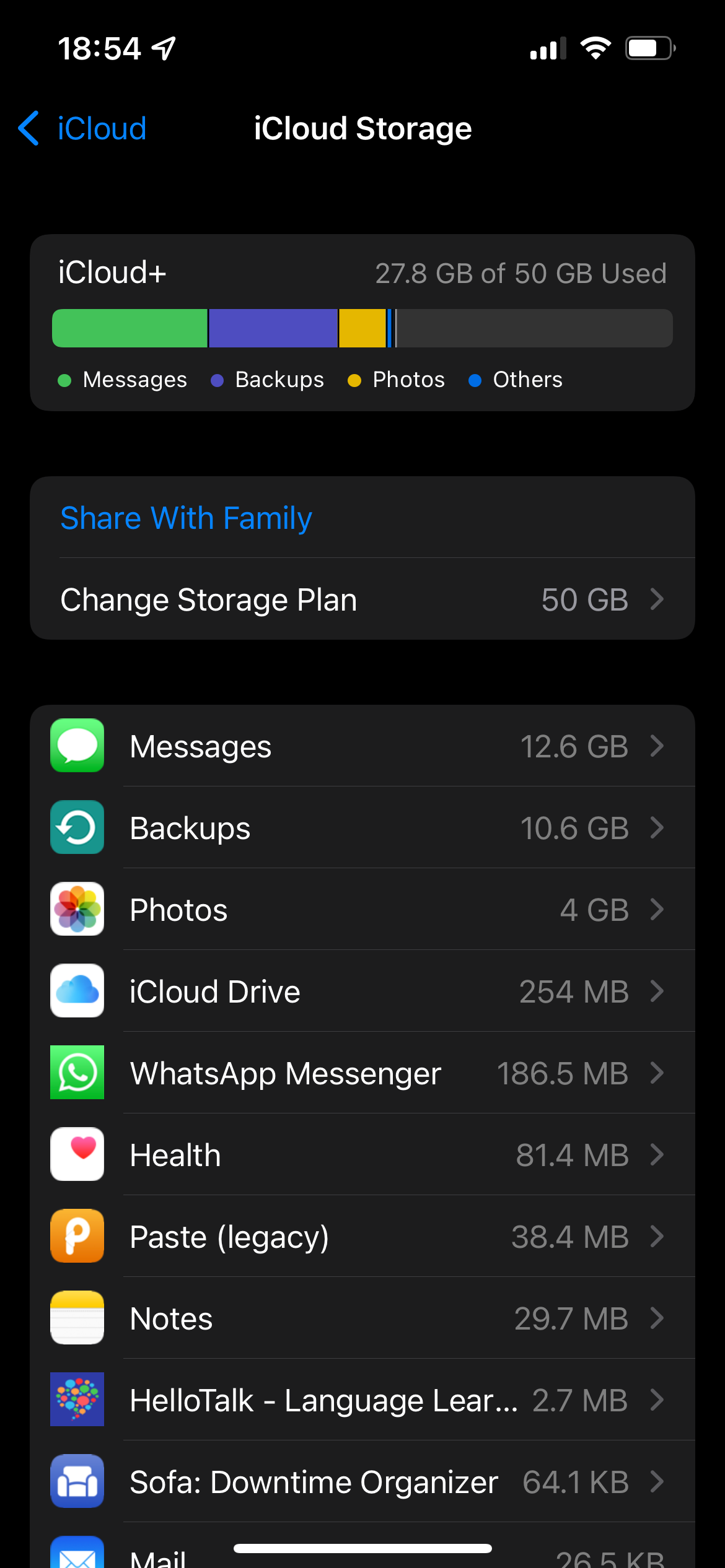This image, captured on an iPhone or tablet, features a predominantly black background. At the top, a blue left arrow with the word "iCloud" points to the previous screen. Centered below it in white text is the title "iCloud Storage." Further down the screen is a white text box labeled "iCloud Plus," accompanied by gray text indicating "27.8 GB of 50 GB used."

Below this information is a colorful horizontal chart displaying the iCloud storage allocation, segmented into different categories. The largest section in green is labeled "Messages," followed by a blue section for "Backups," a yellow section for "Photos," and another blue section labeled "Others."

Below the chart, two rows together display options to "Share with Family" and "Change Storage Plan, 50 GB," each marked with a right arrow.

Further down, a series of rows list various icons and corresponding storage usages:
- Messages: 12.6 GB
- Backups: 10.6 GB
- Photos: 4 GB
- iCloud Drive: 254 MB
- WhatsApp Messenger: 186.5 MB
- Health: 81.4 MB
- Paste (Legacy): 38.4 MB
- Notes: 29.7 MB
- HelloTalk (Language Learn): 2.7 MB
- Sofa (Downtime Organizer): 64.1 KB